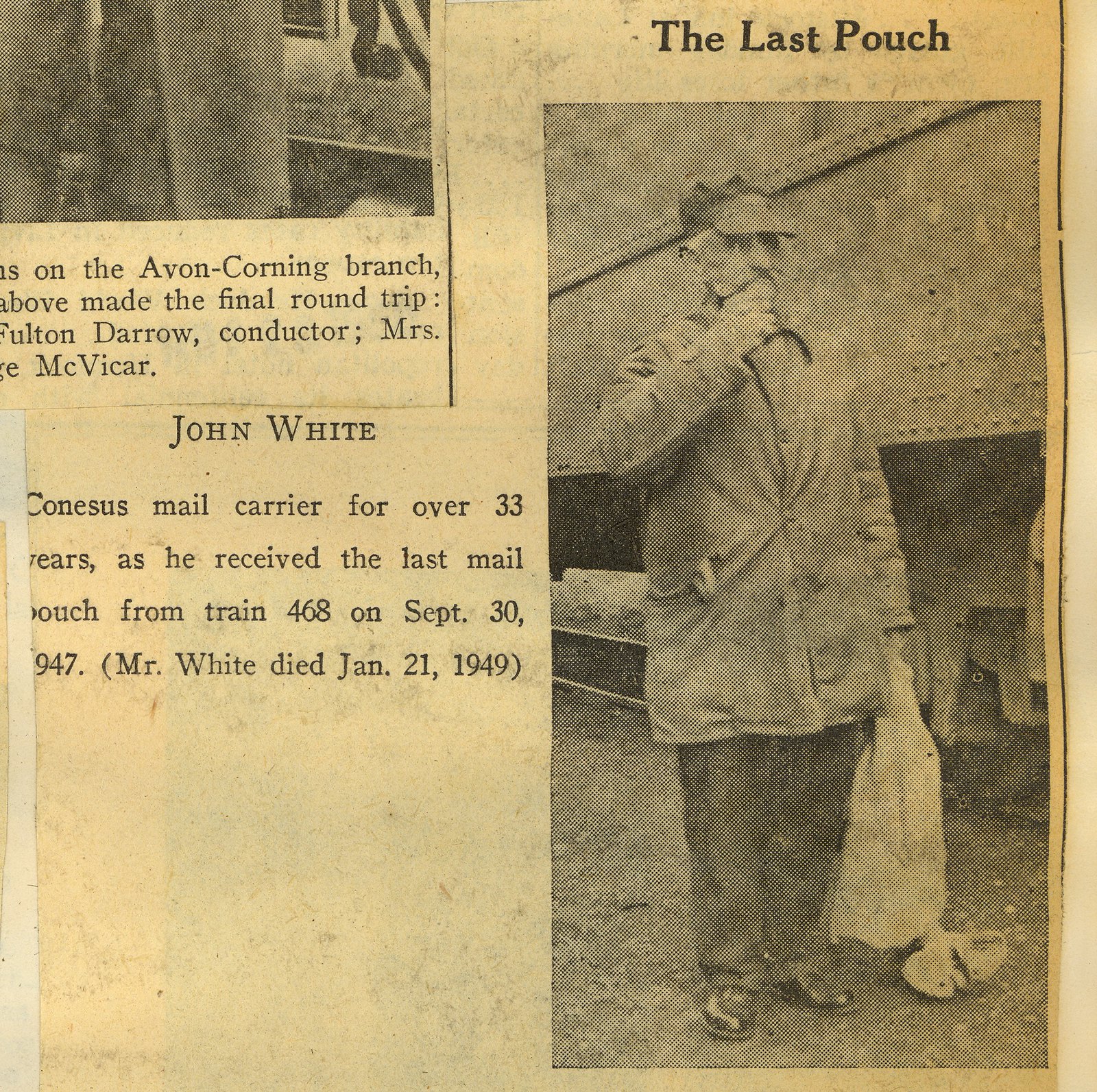The image is a discolored, yellowed newspaper clipping that appears to be quite old. In the upper right-hand corner, the title "The Last Pouch" is prominently printed in bold black letters. Below the title is a black-and-white photograph of an elderly man, John White, who is wearing a baseball cap, glasses, a long coat, and baggy pants. He stands next to what seems to be a train, holding a bag in his left hand and resting his right hand on his chin. Adjacent to the photo, in all capital black letters, are the words "John White." The accompanying text reads, "Connoisseur's mail carrier for over 33 years as he received the last mail pouch from train 468 on September 30th, 1947. Mr. White died January 21st, 1949." The lower left-hand corner of the image contains some bare, brownish newspaper color with small dark brown smudges.